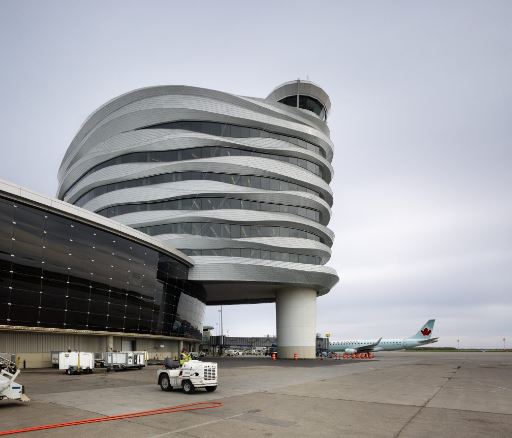This photograph showcases a striking, contemporary air traffic control tower at a modern airport, set against a backdrop of a cloudy sky. The tower, part of a round black glass-windowed building with a curved facade, displays a unique multi-layered design featuring six floors with a waved pattern and large glass windows, topped off by the round structure where air traffic controllers sit, offering them an expansive view. In the background, an airplane is visible on the runway, surrounded by various airport vehicles such as luggage carriers and cargo stations, indicating the bustling activity of loading and unloading luggage. The foreground features a broad, white pedestal-type pillar seamlessly integrating into the main building, emphasizing the airport's modern architecture and design. The scene captures the essence of a busy and advanced aviation hub operating under overcast skies.